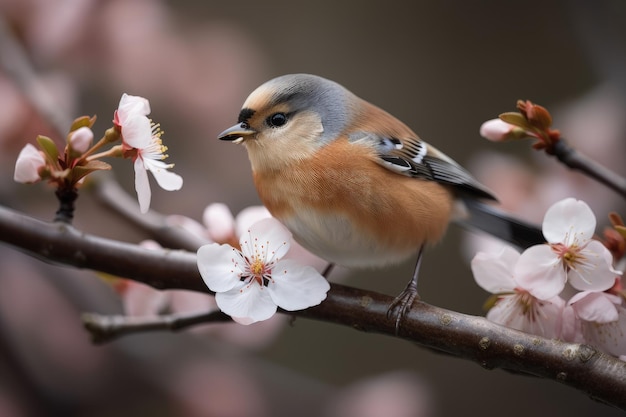In this detailed image, a small, chubby bird perches elegantly on a dark brown, slightly orange-tinted twig adorned with vibrant blossoms. The twig displays a mix of fully bloomed and budding flowers, characterized by white petals with pink and light red centers. The bird, approximately the size of a hand, showcases a predominantly brown body with an off-white, almost beige belly. Its head is a distinct grayish-black with a little black area near the beak. The wings feature black and white stripes interspersed with gray. The shiny twig also holds a shiny branch off to the right, where a flower is just beginning to bloom. In the muted brown background, accented by more pink blossoms, the bird gazes off to the left, capturing a serene early morning or late afternoon atmosphere.